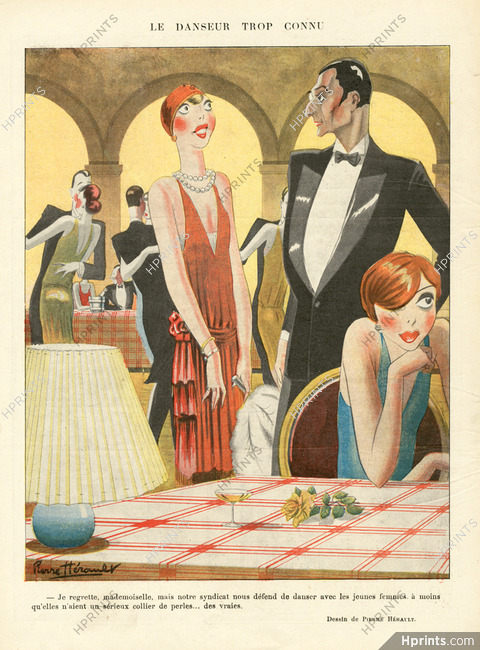The image is a vertically aligned rectangular page with a light tan border or background. At the top, it prominently features the title "LES DANSEURS TROP CONNUS" in all caps, black text centered. Below the title, there's a large drawing in a cartoonish vintage French art style.

The focal point of the drawing is a very slender woman in an orange sleeveless dress with ruffles at the bottom. She has two strands of pearls around her neck and an orange wrap matching her dress in her hair. She is smiling broadly, with noticeable red lipstick, at a man in front of her who is dressed in a tuxedo and has short black hair. 

In the lower right corner, a second woman with short red hair sits at a table, resting her chin on her hand. She is wearing a blue sleeveless dress. Notably, there is a lamp on this table with a round blue base and a long lampshade.

The scene is lively, with additional figures in the background, dancing in front of arched windows. Another distinctive feature of the table is its red and white checkerboard design. The entire drawing has a watermark with the letters "H-Prince" across it. At the bottom of the drawing, there are two lines of text in French, along with an illegible signature in black ink in the lower left corner.